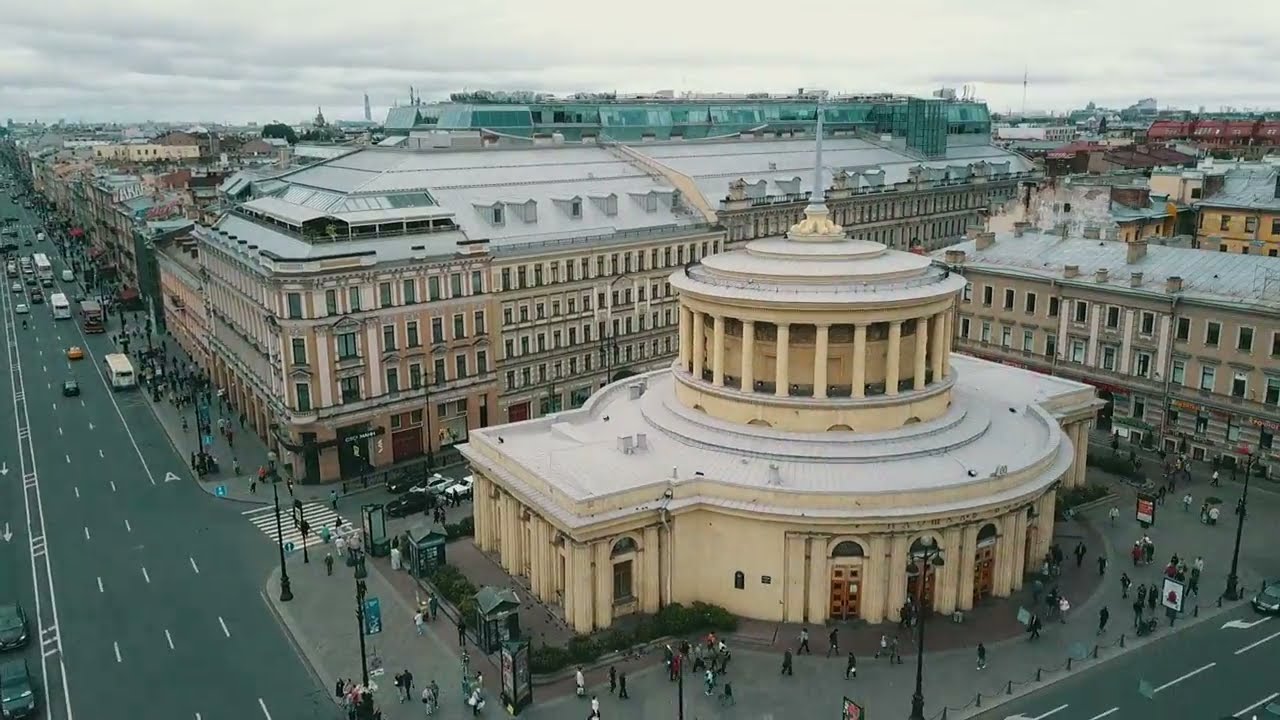This photograph captures a bustling urban scene centered around a prominent cream-colored, two-story building with a green metal roof and dark, rectangular windows. The structure prominently features a central tower capped with a green dome, housing a circular analog clock on its second story, with an antenna extending from its peak. The facade of the building displays foreign wording, "M-O-C-K-O-B-C-K-N-N" and "B-O-K-E-A-J," in white letters outlined in green.

In front of the building is a walkway teeming with people dressed predominantly in dark clothing. Below the walkway lies a busy street and a fully occupied parking lot featuring a variety of vehicles, including a noticeable yellow taxi cab and a light red car vying for space. The skyline in the distance reveals a tightly packed array of buildings, suggesting a dense urban environment. The sky above is overcast with a mix of gray and white clouds, allowing only minimal light to filter through, casting a somewhat dark and hazy ambiance over the scene. Overall, the image suggests a lively and crowded city area.